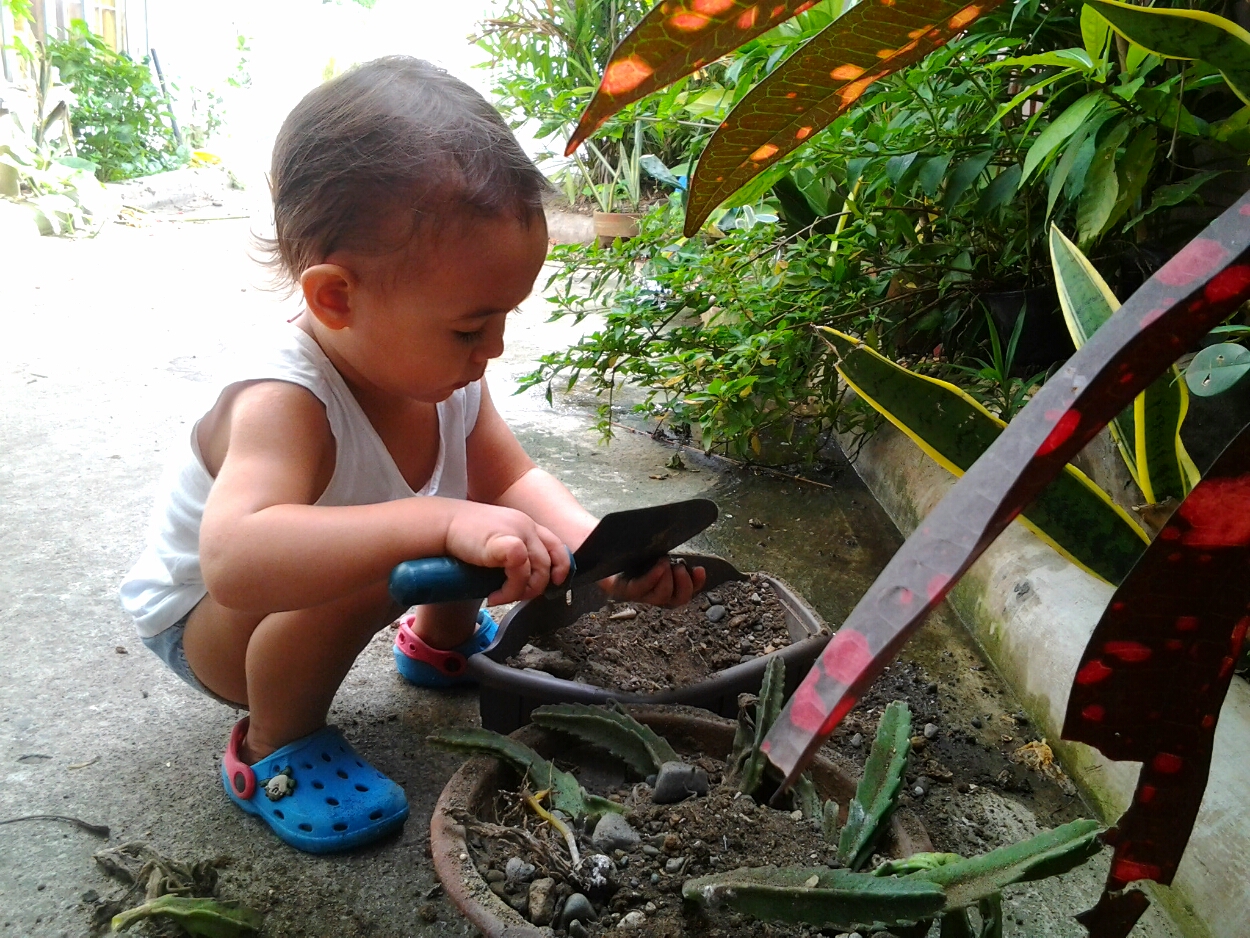This photograph captures a young child, approximately two years old, engaging in gardening activities outside. The child, who has dark hair and is wearing a white sleeveless t-shirt and little gray shorts, is squatting on a concrete pathway, clad in bright blue Crocs with red stripes. Using a small blue-handled gardening shovel, the child is diligently transferring gravel from the ground into their left hand and a nearby pot. This pot once held a Christmas cactus, now uprooted with remnants scattered around. Surrounding the walkway, lush tropical plants create a vibrant backdrop, featuring red and green, green and yellow foliage, snake plants, and various vines. The setting behind the child includes abundant greenery and a neatly maintained garden area adorned with bushes and shrubs. A larger potted plant with green vegetation and a protruding garden tool with a long black handle can be seen nearby, adding to the scene of outdoor exploration and learning.